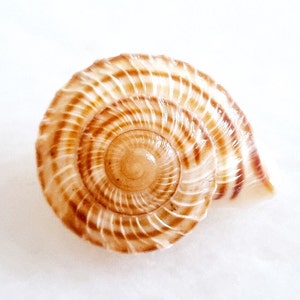This is a detailed drawing of a spiraled seashell, specifically resembling the shape of a nautilus or a snail shell. The shell is primarily round, featuring a series of intricate spirals that swirl clockwise towards the center, where it terminates in a smooth, light brown area. The shell is adorned with multiple bands of colors ranging from dark brown to light brown and cream, enhanced with white, ribbed ridges that add a rough texture to the exterior. The ridges, raised and primarily white, accentuate the shell's swirling pattern. There are six to eight distinct swirls from the top to the bottom, where they converge.

The shell opens widely on one side into a fluted aperture, which is where the snail or creature could emerge. This opening is banded with the same earthy tones, creating a consistent aesthetic across the entire shell. The background highlights the shell's features, as it is a pale, off-white color, making the shell's detailed banding and textured ridges stand out. The image presents a harmonious blend of symmetry and organic growth, capturing both the artistic representation and the natural beauty of the shell.